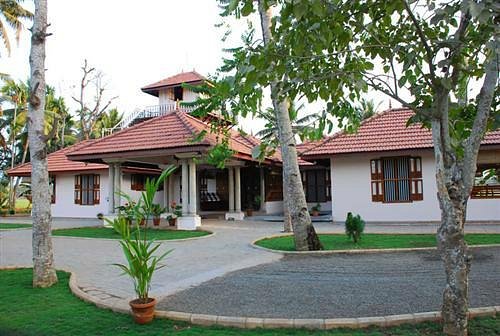This image captures the expansive facade of a large white stucco house with distinctive red Spanish tile roofing, featuring an orangish-reddish hue. The structure includes a prominent tower at the back left, also adorned with the same red tile roof. The central portion of the house showcases wide glass doors beneath a canopy supported by white concrete columns, providing a shaded area for unloading vehicles. The driveway, divided into two intertwining sections, is bordered by meticulously manicured green grass, gray pebbled stones, and several lush trees, including palm trees in the distance. The windows, some framed with brown wooden shutters and bluish blinds inside, punctuate the white walls. In front of the house, a pot of long green leafy plants adds to the verdant, well-maintained landscape. Above, the sky is a clear blue dotted with some clouds, framing the picturesque setting.